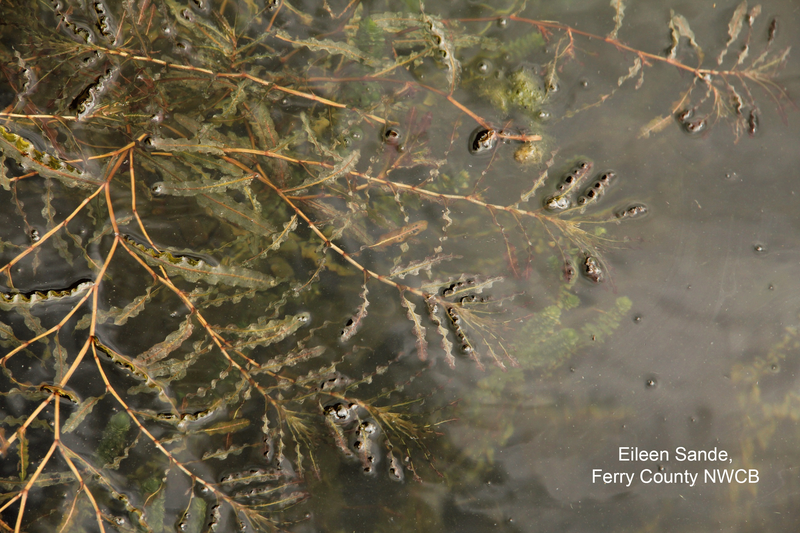The image depicts an outdoor scene of an evergreen tree partially submerged in brackish, slightly hazy water. Thin, brownish-beige stems and green needle-like leaves of the evergreen are visible amidst the water, which also exhibits some bubbles suggesting possible aquatic life. The photograph, which has a horizontal rectangular format, features a heavy shadow on the right side. In the bottom right corner of the image, white text reads, "Eileen Sand, Ferry County, NWCB."